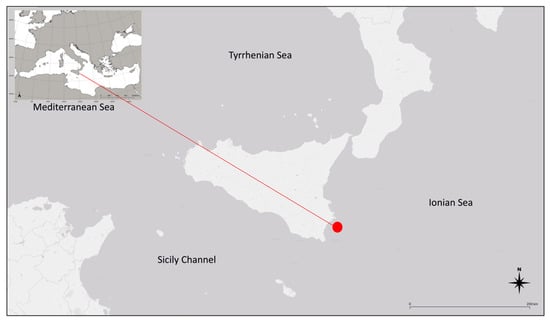This detailed black and white map of the Mediterranean Sea focuses on the lower half of Italy and Sicily, with one prominent red line drawing attention to specific locations. The surrounding ocean waters are depicted in a light gray color, while Italy, Sicily, and other adjacent lands are in white. Key parts of the sea are labeled in black, including the Ionian Sea to the right, the Sicily Channel to the south of Sicily, the broader Mediterranean Sea, and the Tyrrhenian Sea to the north. The bottom right corner features a compass with a star indicating north. An inset map in the top left corner provides a wider view, pinpointing the specific area detailed in the larger map.